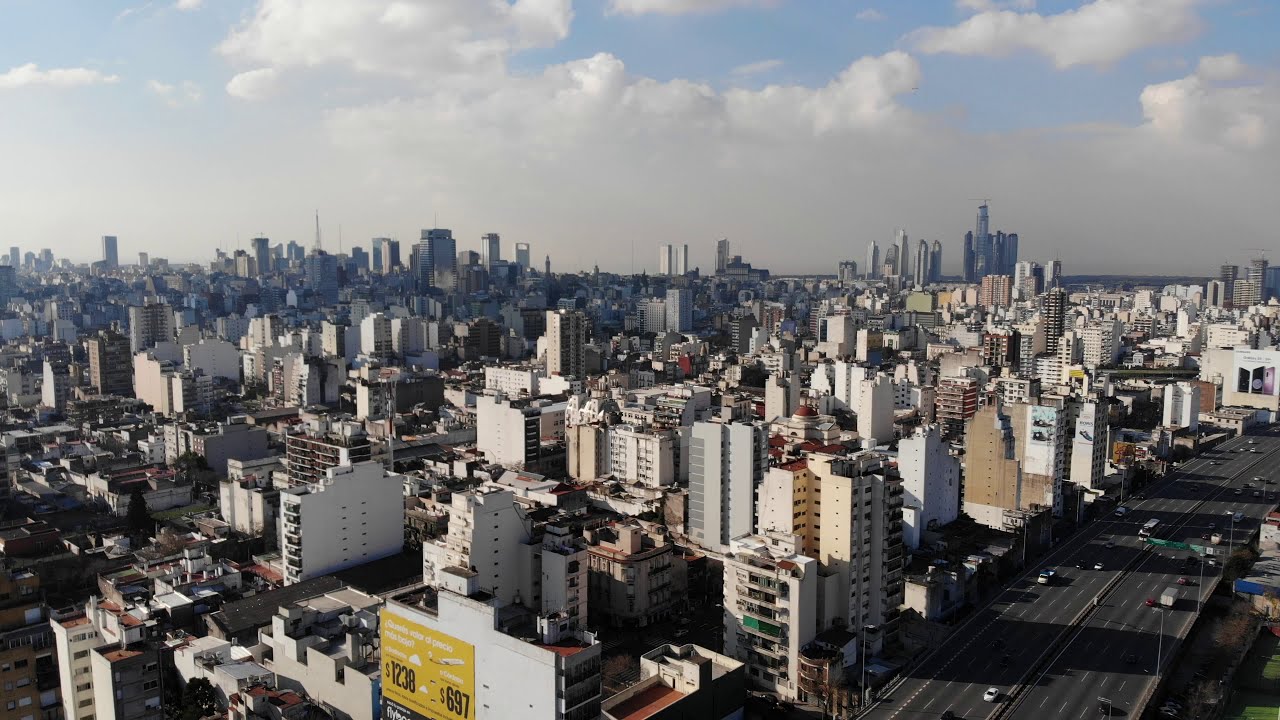An expansive aerial view of a bustling metropolis showcases numerous high-rise buildings spanning from the left to the right edges of the image, with no greenery in sight. Prominent in the distance are two towering structures that strongly resemble the Twin Towers, suggesting the cityscape of New York City. In the foreground, a major eight-lane highway cuts diagonally across the bottom right corner, teeming with a variety of vehicles including a noticeable white semi-truck amid smaller cars in black and white. Adjacent to the highway is a white building adorned with a striking yellow billboard displaying the numbers "$1238" and "$697" in white text. The skyscrapers vary in height, typically between 8 and 15 stories, with some shorter buildings interspersed among them, especially towards the left side. Further into the distance, the skyline ascends into even loftier structures under a backdrop of white clouds and a serene blue sky.